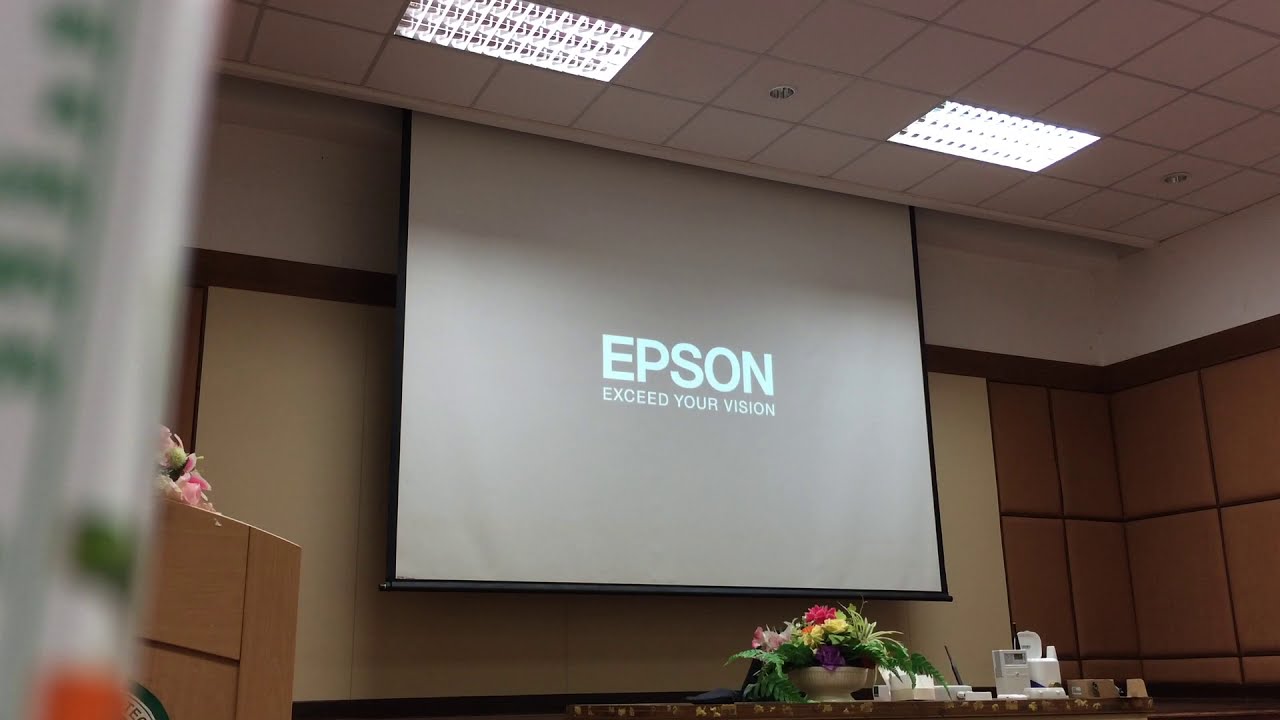The image depicts a meticulously arranged conference room, possibly within an office or a hotel. Dominating the scene is a large projector screen descending from the ceiling, prominently displaying "Epson: Exceed Your Vision." The ceiling features well-integrated lighting and is tiled with white squares, creating a bright and professional atmosphere. The wall behind the projector screen is beige, contributing to a warm, inviting ambiance. In front of this wall is a table adorned with a flower vase and assorted stationery, adding a touch of elegance and practicality. To the side of the table, a partially visible dais suggests the presence of a speaker, indicated by the arrangement of flowers on it. No other people are present in the image, highlighting the room’s setup and readiness for an upcoming presentation or meeting.